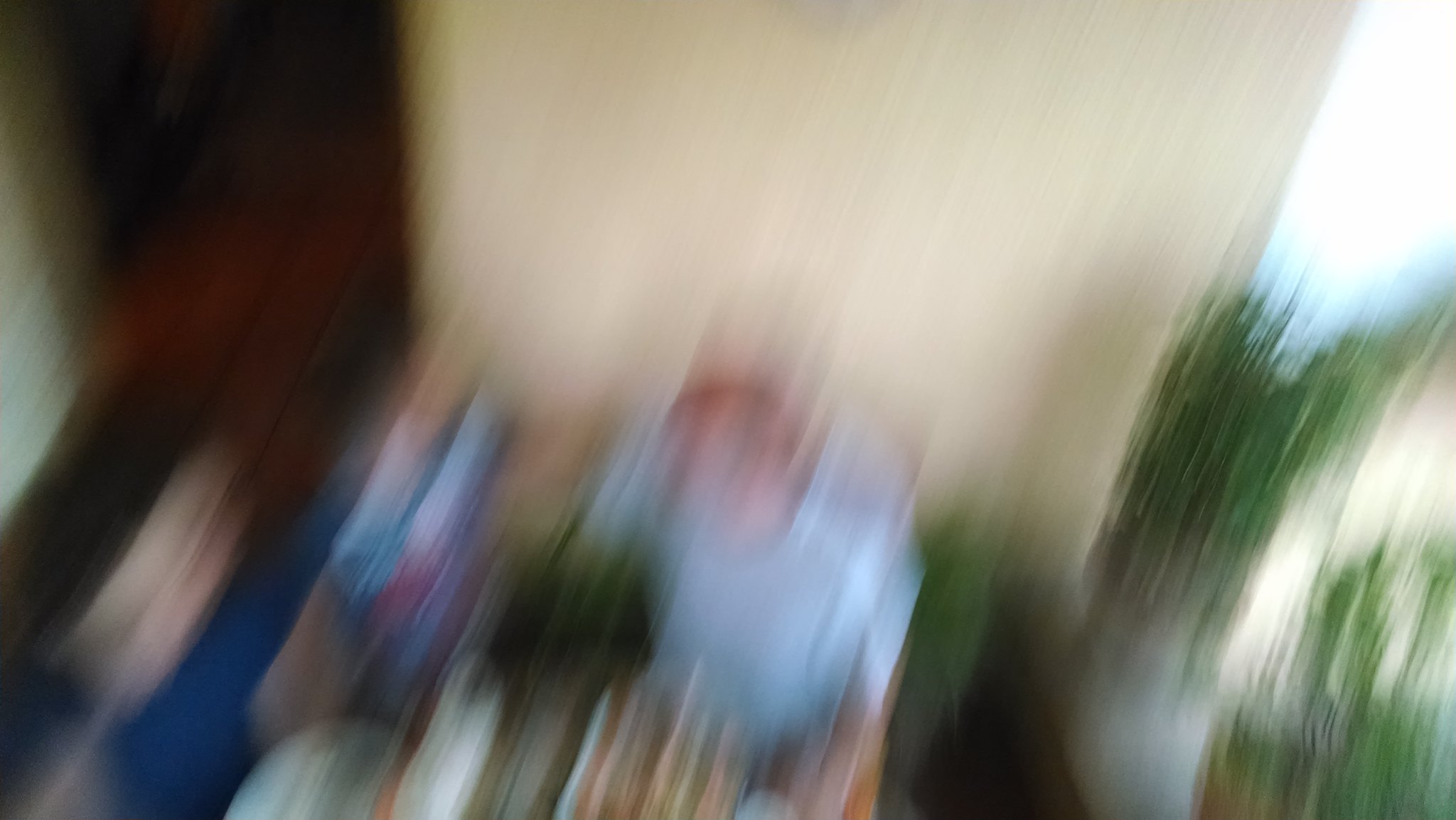In the slightly blurred photograph, two individuals are seated inside a building with a white wall as the backdrop. On the right side of the image, there appear to be green elements, possibly trees or plants, visible through an adjoining window or a partially open door. The first individual, located on the right, is a male with Caucasian skin, dressed in a white short-sleeved shirt and possibly orange-colored pants or shorts. To the left, a female with dark hair is wearing a blue short-sleeved top. Both subjects seem to be sitting at a table, though details of the table itself are obscured by the blur.